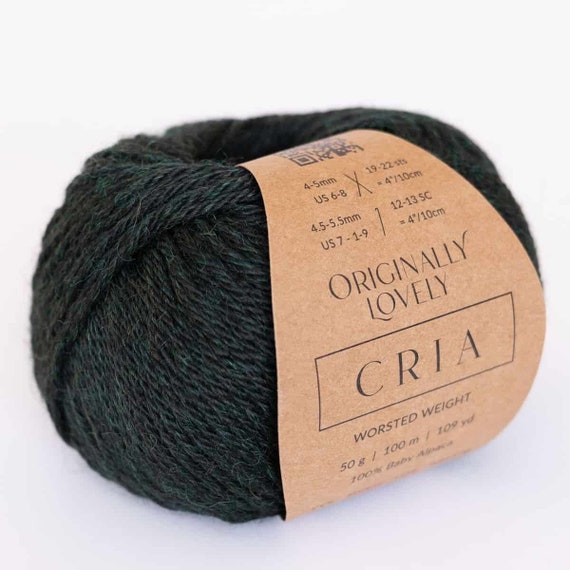This image depicts a neatly packaged skein of yarn, predominantly dark gray, almost black, interwoven with subtle greenish hues. The yarn, which looks brand new and is tightly wrapped, has a tan label made of what appears to be a cardboard-like material. The label contains black text, detailing that the yarn is named "Originally Lovely CRIA" and is of worsted weight, indicating the thickness of the material. It is composed of 100% baby alpaca, weighing 50 grams with a length of 100 meters (109 yards). The label also includes a QR code at the top, information about needle sizes (4-5 mm U.S. 6-8, 4-5 to 5.5 mm U.S. 7-9), and a stylishly written text. The overall shape of the skein is slightly oval and is slightly tilted to the left against a plain white background.